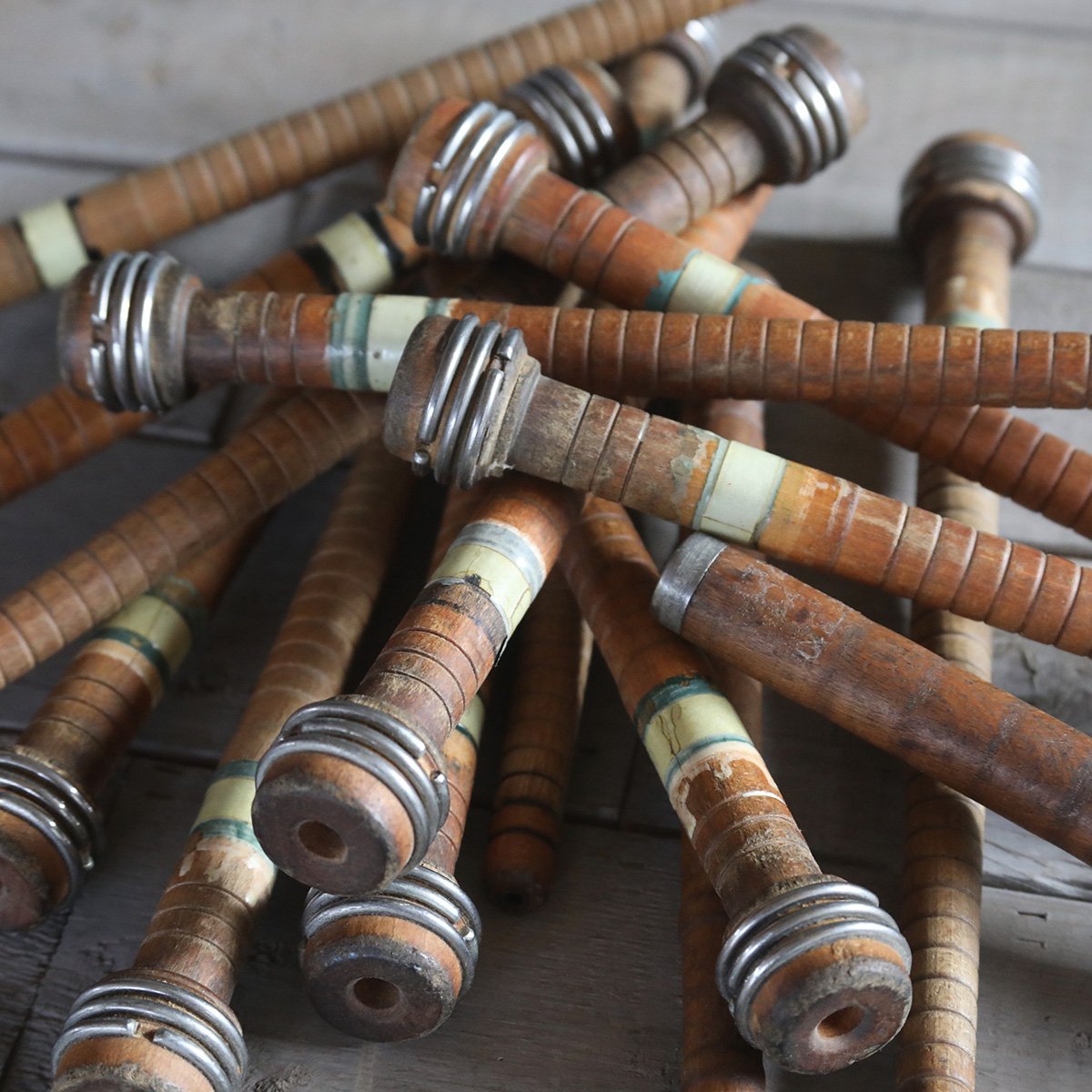This square-shaped color photograph, taken indoors with artificial lighting, captures a small pile of antique wooden spools or bobbins resting on a wooden workbench. The spools are arranged in a random pattern, with approximately twelve visible, each made of wood varying in color from rich red brick to golden hues. These wooden spools feature smooth sections with notches or circular rings and have silver wire wrapped around their tops three times. At the top of each spool is a round hole. Some spools bear faded labels with green and yellow lines, adding to their vintage charm. While a few spools in the top left corner are out of focus, the overall composition showcases a sense of nostalgic realism.